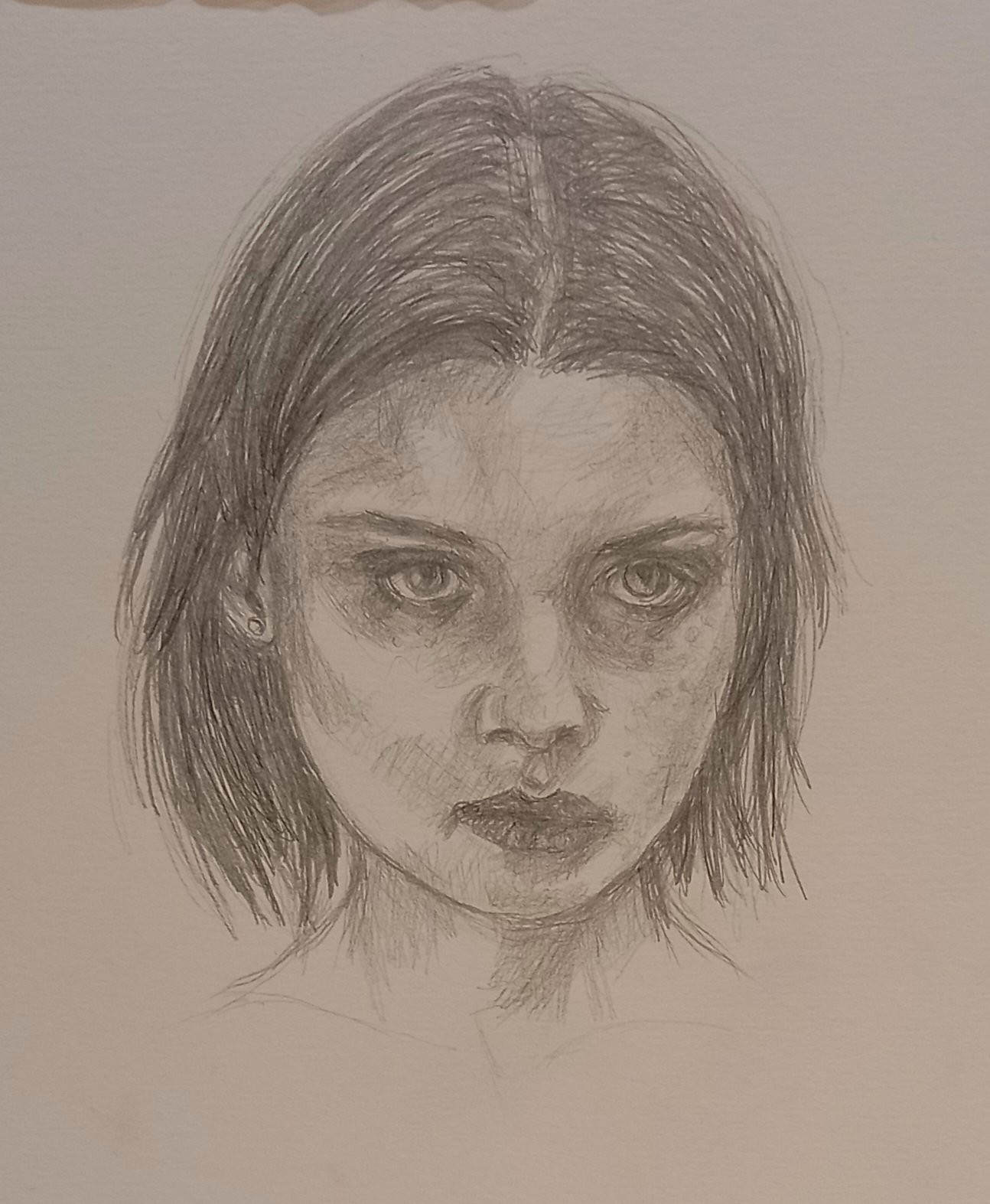This drawing, likely done in pencil on off-white paper with a pinkish tint, presents a detailed portrait of a woman. Central to the composition is her face, framed by shoulder-length hair parted down the middle. The woman's expressive eyes, exhibiting a look of fatigue with noticeable dark circles underneath, dominate her delicate features. Her right ear, adorned with a stud earring, peeks through her hair. Her nose is small and cute, while her full lips add to the richness of her expression. The woman's head is directed slightly to the right of the viewer, and her overall demeanor suggests an air of melancholy or pensiveness.